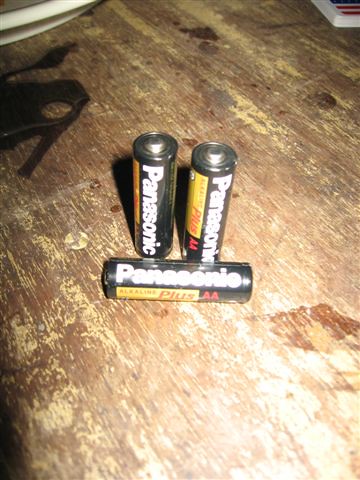This photo depicts three Panasonic Plus AA batteries placed on an old, worn wooden table. Two of the batteries are standing vertically, side-by-side, while the third one lies horizontally in front of them. All three have a black background with the Panasonic logo prominently displayed in white, accompanied by a red "Alkaline Plus" label on a yellow strip, and the "AA" designation in red. The tabletop itself shows significant signs of wear, with scratches, stains, watermarks, and dark spots, along with a noticeable wet area close to the horizontal battery. In the top left corner of the image, the edge of what appears to be a white dinner plate is faintly visible.